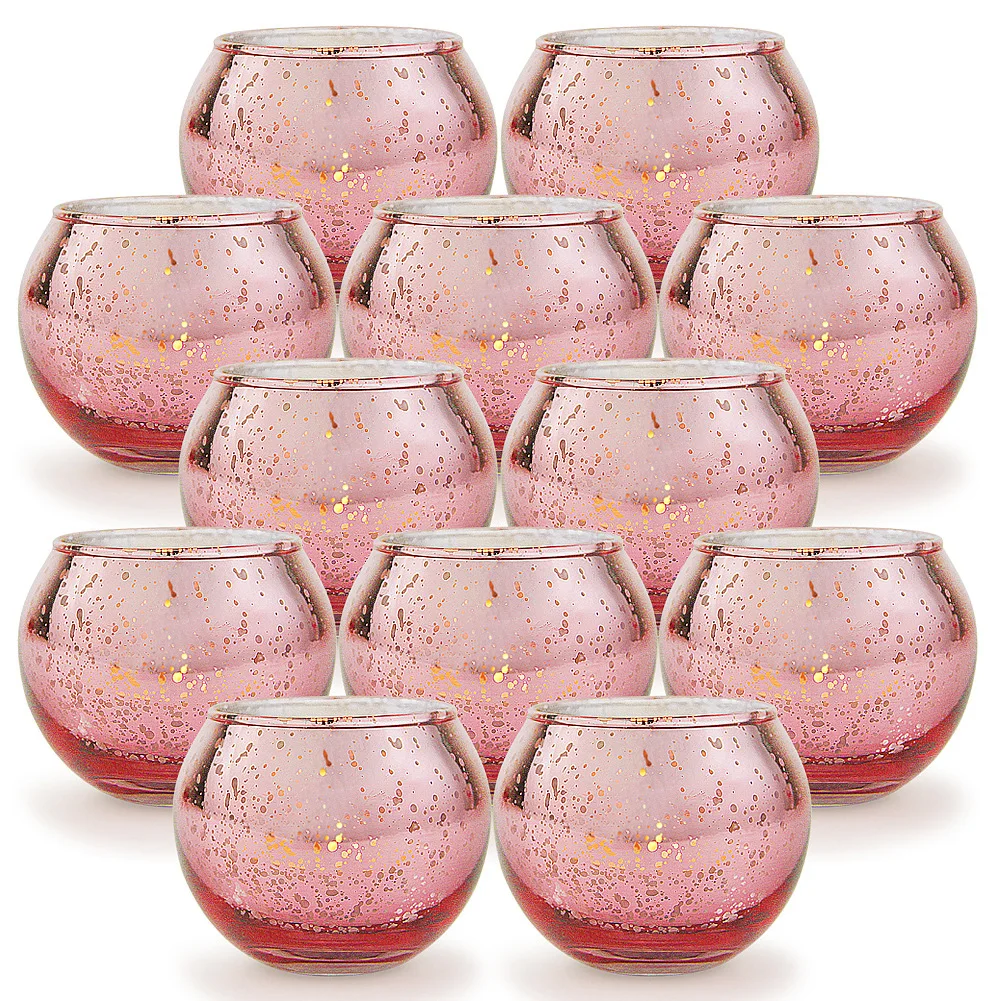The image depicts a meticulously arranged 12-piece set of round glass votive candle holders, displayed on a clear white background. Each candle holder is crafted from glass and features a light pink hue adorned with gold speckles. These delicate speckles and spots add an elegant touch, shimmering subtly against the glass. The pink coloration fades into a slightly darker shade towards the base, creating a gradient effect. They are organized in a staggered manner, forming rows of two, three, two, three, and two, almost resembling a pyramid shape. Shadows below each holder indicate a slight elevation, possibly due to the transparency of the glass. Ideal for home decor, weddings, or festive occasions like Christmas, these candle holders are designed to accommodate tea light candles, creating a charming and sophisticated visual appeal.